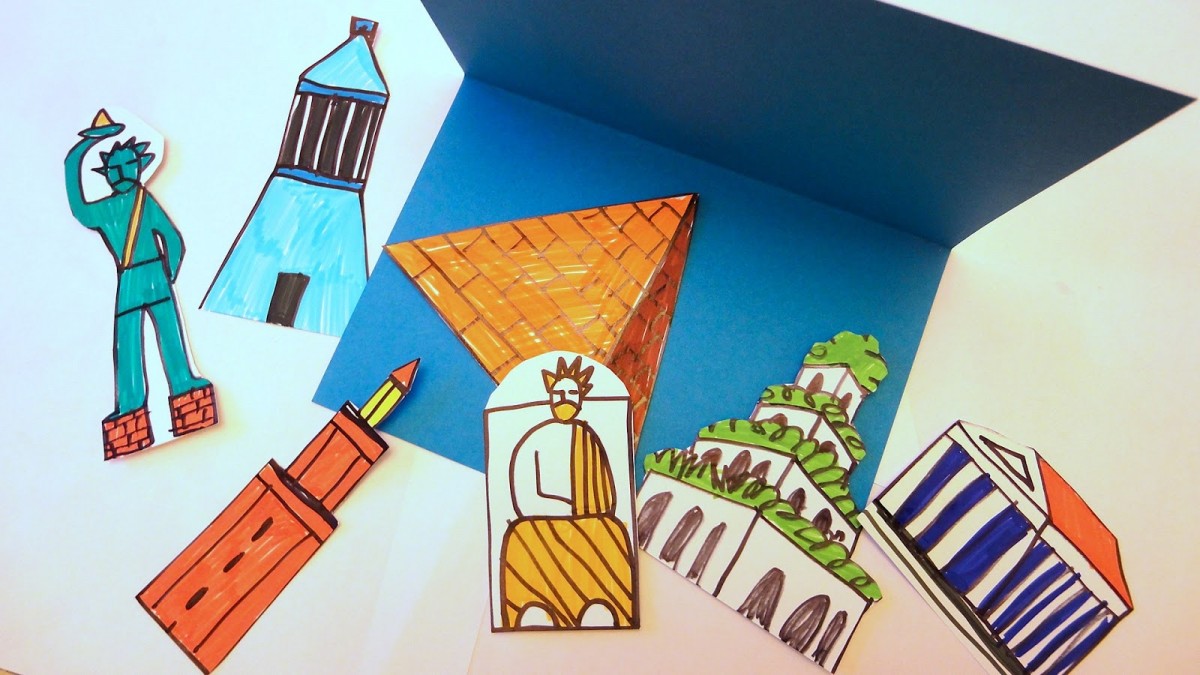The image features an open, bright blue greeting card, positioned on a white backdrop. Arranged around it are various rudimentary, hand-drawn paper cutouts of famous monuments and landmarks, each colored in vibrant hues. Notable among these are the Statue of Liberty holding a safari hat, the Great Pyramid of Egypt, the Colosseum, the Parthenon, perhaps the Tower of Babel, Big Ben, the Hanging Gardens of Babylon, and a figure resembling Zeus. These landmarks, representing the Seven Wonders of the World, are scattered both inside and around the greeting card, giving an impression of global exploration and admiration for architectural marvels.